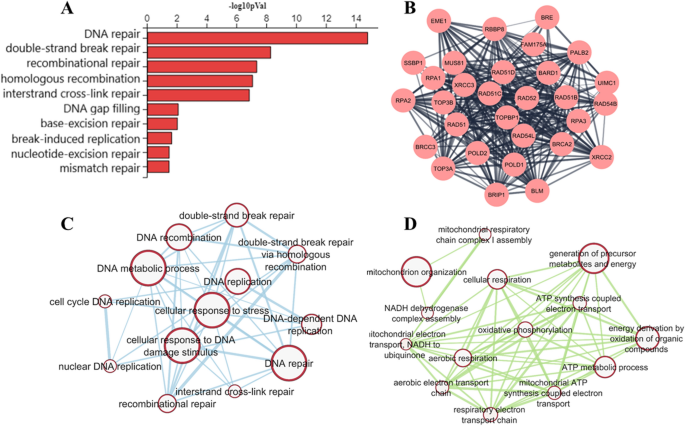This image consists of four distinct diagrams labeled A, B, C, and D, elaborately detailing various aspects of DNA repair mechanisms and processes. 

In the top left (A), a horizontal bar graph with red bars illustrates different DNA repair pathways. The vertical axis lists processes such as DNA repair, double strand break repair, recombinational repair, homologous recombination, interstrand cross-link repair, DNA gap filling, base excision repair, break-induced replication, nucleotide excision repair, and mismatch repair. The horizontal axis ranges from 0 to 14, quantifying the instances or activities related to these processes. 

Adjacent to it in the top right (B), there is a complex network diagram resembling a kaleidoscope or spider web, composed of numerous pink circles interconnected by black lines. Each circle contains black text identifiers such as RPA1, TOP3B, BLM, and XRCC2, which likely represent various proteins or genetic markers involved in these repair pathways.

The bottom left (C) features another network diagram similar to B, but with red circles that have white centers. This diagram also contains numerous light blue connecting lines and labels for processes like double strand break repair, DNA metabolic process, and nuclear DNA replication, indicating interactions and pathways within these processes.

In the bottom right corner (D), yet another web-like network is displayed, this time with light green lines and more red circles with white centers. Labels within the circles include terms like oxidative phosphorylation and mitochondrion organization, suggesting a focus on metabolic and cellular organization processes related to DNA maintenance and repair.

Together, these diagrams provide a detailed and interconnected view of DNA repair mechanisms, emphasizing the complexity and interrelation of various genetic processes.